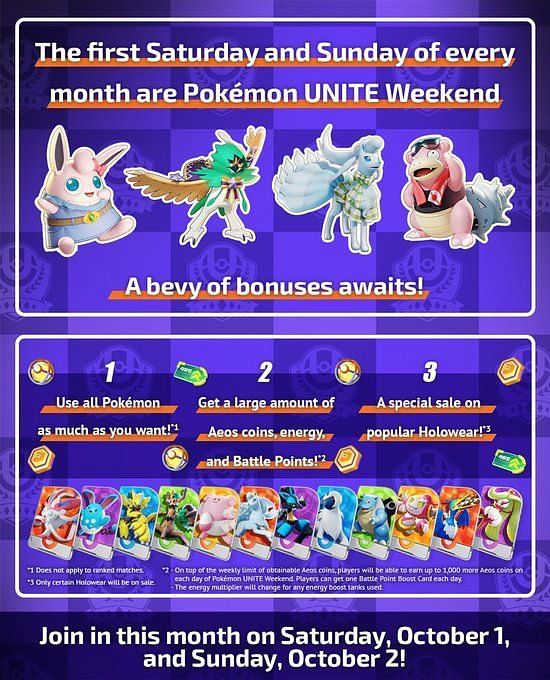Caption: 

An intricately detailed promotional sign announces "Pokemon Unite Weekend," celebrated on the first Saturday and Sunday of each month. Prominently featured are four diverse Pokémon characters: a small pink rabbit-like Pokémon, a green headdress-wearing Pokémon with gold wings and clawed feet, a majestic blue variant of Ninetales with multiple tails, antlers, and ears, and a pink and tan Pokémon with a bite mark on its rear. The vibrant text in white set against an orange shelf background proudly declares, "A bevy of bonuses awaits."

The backdrop showcases a light and dark purple checkerboard pattern adorned with Pokéballs in the dark squares. Centered within a white box are details about the weekend's special features:
1. Unlimited usage of all Pokémon
2. Generous rewards of AEOS coins, energy, and battle points
3. Special sale on popular holoware

Below these features, 12 different Pokémon are spotlighted on individual cards. The fine print at the bottom emphasizes that the bonuses do not apply to ranked matches, players can earn an additional 1,000 AEOS coins each day of the weekend, a battle point boost card is available each day, and energy multipliers will be adjusted for any energy boost tanks used.

In a bold black rectangle at the bottom, the call to action reads: "Join in this month on Saturday, October 1st and Sunday, October 2nd."